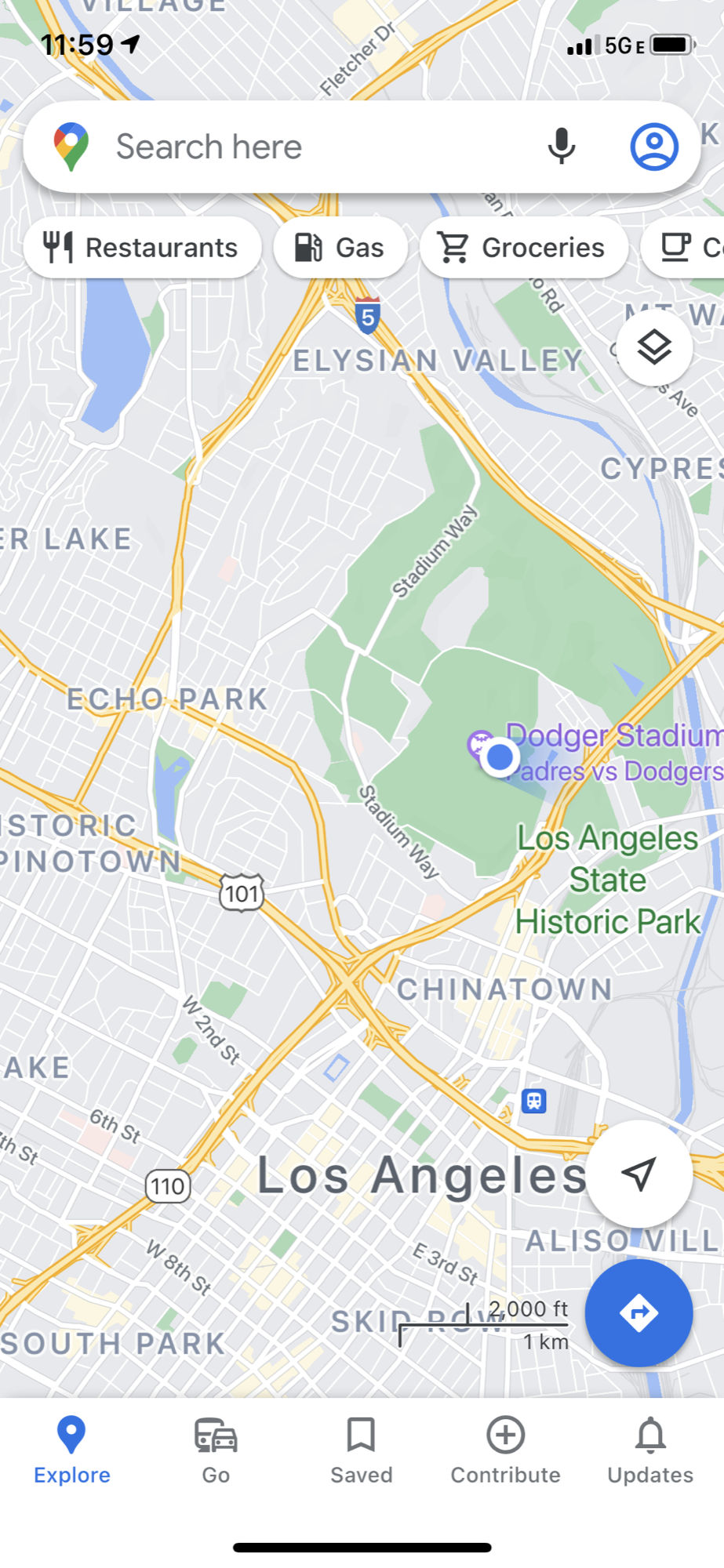This photo captures a smartphone screen displaying a navigation application with a detailed map of Los Angeles. At the top of the screen, the time is shown as 11:59, alongside indicators for a 5G network connection, battery percentage, and other status icons. Below this, a Google search bar is prominently featured, with a microphone icon and the text "Search here," suggesting that the user can perform voice searches. Beneath the search bar are shortcut buttons for locating nearby restaurants, gas stations, grocery stores, and other amenities, although not all options are visible.

The central part of the screen is dominated by a map highlighting several key locations in Los Angeles, including Echo Park, Chinatown, Dodger Stadium, Los Angeles State Historic Park, and Elysian Valley. At the bottom of the map, various navigational and interactive icons are present. There is a centered, solid blue arrow pointing upwards, flanked by a white button to its right and a white arrow in a black circle pointing towards the top right corner of the screen. Additionally, there are tabs for exploring more options labeled "Explore," "Go," "Save," "Contribute," and "Updates."